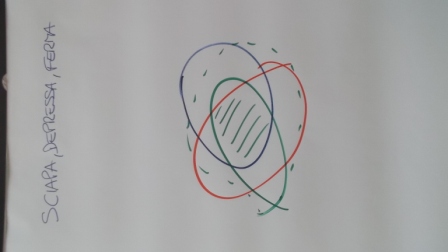This is an image of a whiteboard that has been rotated to the left, making the original top of the board appear on the left side of the photo. On what is now the left edge, there is a series of handwritten, capitalized words in either black or dark blue ink. These words are "SCIAPA," "DEPRESSA," and "FERMA," written in a somewhat messy manner.

In the right-center of the image, there is a diagram composed of three distinct colors. First, there is a roughly sketched solid orange circle. Overlapping parts of this circle is a green shape, which appears to be an X made of circles. The green shape is thin and similarly haphazardly drawn. Additionally, a blue circle overlaps half of the green X, and the green X intersects parts of the orange circle. Among these shapes is a blue dotted line circle that intersects through the center of all the other circles, creating an interconnected, yet chaotic, visual design.